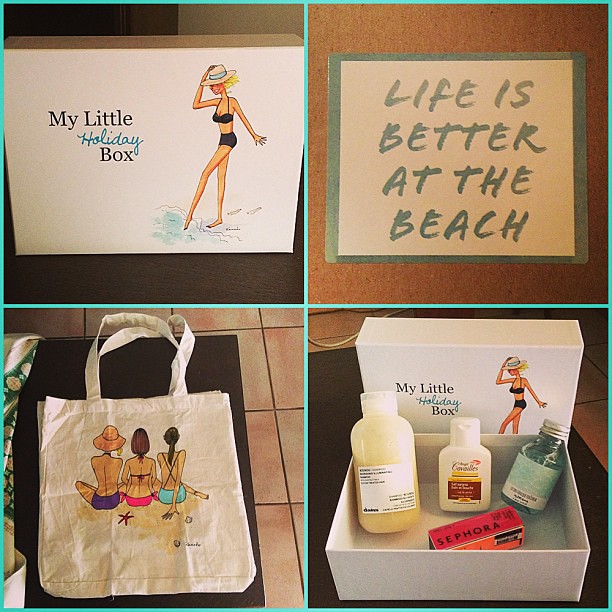This image is a detailed compilation divided into four square sections, bordered by an intersecting aqua-colored frame. The top left section features the top cover of a white box with the text "My Little Holiday Box" prominently displayed. To the right of the text is an illustration of a woman in a black bikini with yellow hair, wearing a top hat, and dipping her left foot into the water. The top right section captures a sign with a cream-colored background and silver-toned handwritten text that reads "Life is Better at the Beach." The bottom left section showcases a white beach tote bag lying on a black surface. The bag's graphic depicts three women sitting side by side, facing away from the viewer, at the beach. Finally, the bottom right section displays an open box with three products inside, with the lid visible behind them. The overall style of the image combines photographic realism with graphic design elements, creating a cohesive and vibrant representation of holiday-themed items.